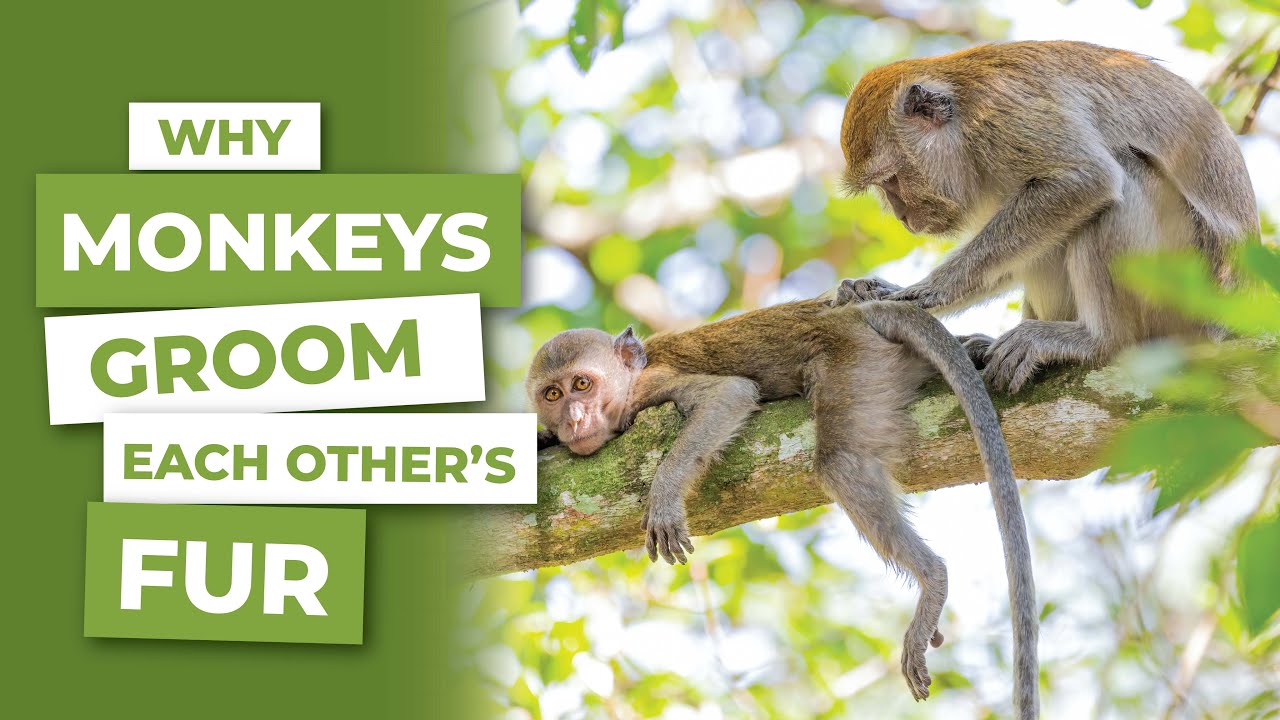This is a two-panel thumbnail for a YouTube video about why monkeys groom each other's fur. On the left panel, there is stylish green and white text layered in block capitals, reading "Why Monkeys Groom Each Other's Fur." The text is set against a dark green background that seamlessly transitions into the right panel. The right panel features a photograph of two grey monkeys with darker russet tones on their backs, perched on a tree branch. One monkey, younger and smaller, lays face down on the branch with its limbs and tail hanging loosely, staring directly at the camera. The other monkey, larger in size, is crouched meticulously over the first monkey, grooming its fur. The background is a blur of foliage and sunlight, placing the primary focus on the interaction between the two monkeys.